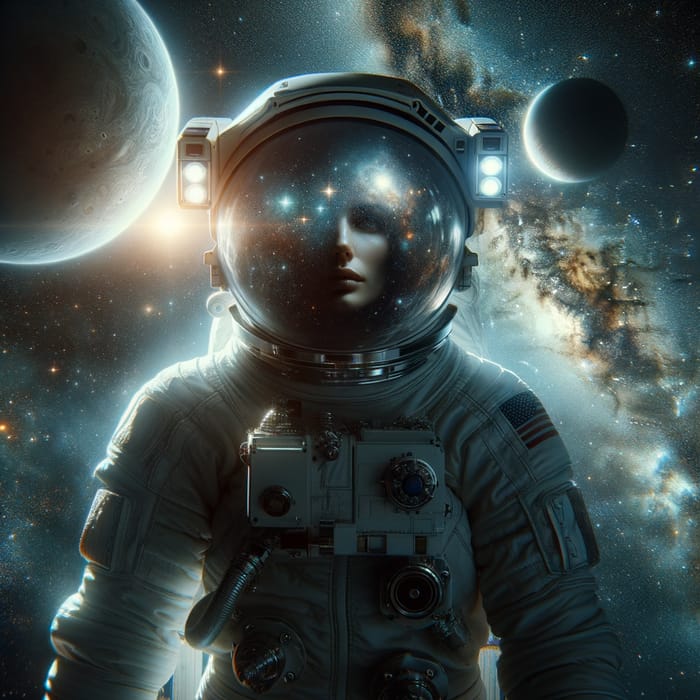A dynamic image captures an astronaut from the torso up, dressed in a full space suit. The helmet visor reveals the face of a woman, although only the left side is visible due to the angle. The remaining visible part of the helmet reflects the vastness of space, showcasing a mesmerizing array of stars and distant galaxies. The backdrop extends this celestial theme, with what appears to be the Milky Way galaxy sprawling magnificently behind her, dotted with countless stars. In the upper right corner above her head, a large planet looms, adding depth to the cosmic scene. To her immediate left in the background, a smaller planet is also visible, further enhancing the otherworldly atmosphere of the image.